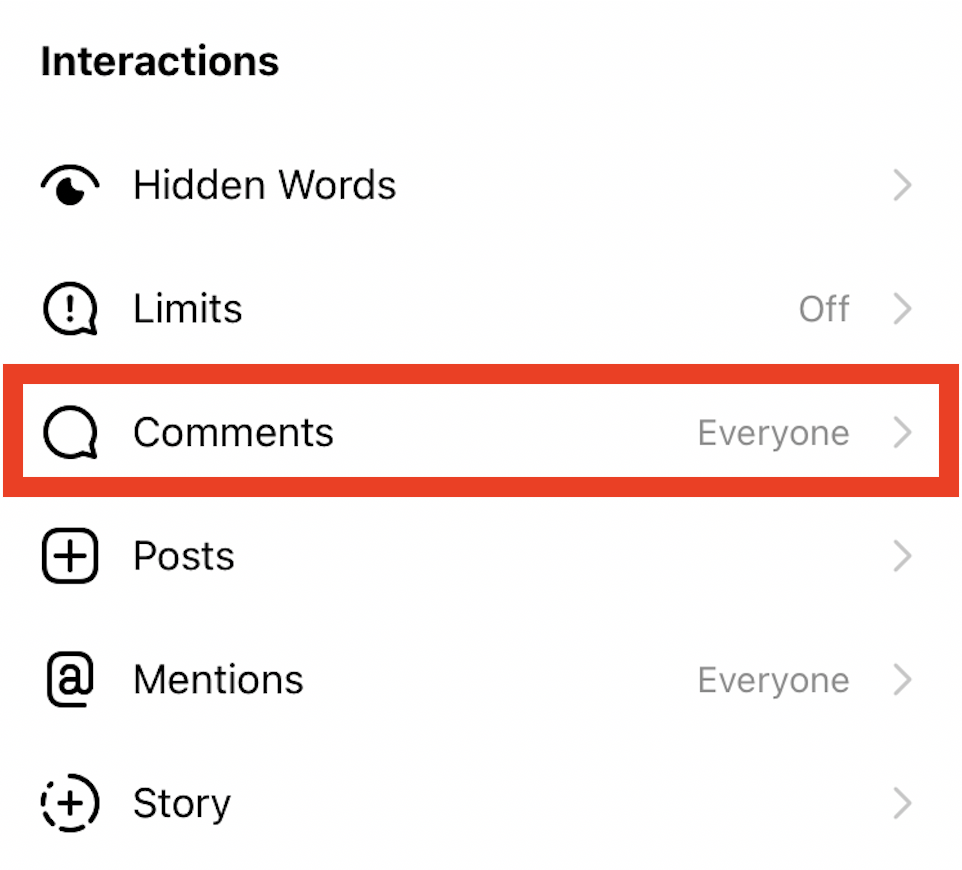This is a detailed view of the interactions settings section within the Instagram app. The cropped screenshot showcases the options available under 'Interactions,' displayed prominently at the top left in bold black font. Below this heading is a vertical list of settings categories. The first option is 'Hidden Words,' accompanied by a right-pointing arrow, indicating additional settings are available for further customization. Following this is 'Limits,' which is currently set to 'Off.' Next is 'Comments,' showing that comments are allowed from 'Everyone.' A prominent red box highlights the 'Comments' section, instructing users to click this option to enable comments from everyone. Beneath 'Comments,' the list continues with 'Posts,' which features an arrow to the right for accessing extended settings. 'Mentions' follows, set to allow mentions from 'Everyone.' Lastly, the 'Story' option also has a right-pointing arrow, suggesting further settings customization. The screenshot is set against a clean, white background, with only the interactions settings displayed, omitting the rest of the app's interface.